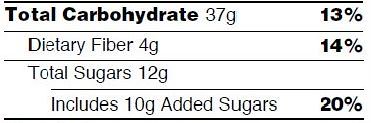This image displays a close-up section of nutritional information, presented in a stark black-and-white color scheme with a white background and black text. The text is divided with black lines, featuring a thicker line at the top and bottom and thinner lines in between. The nutritional facts listed include "Total Carbohydrate 37 grams (13%), Dietary Fiber 4 grams (14%), Total Sugars 10 grams, and 10 grams of Added Sugars (20%)". The term "Total Carbohydrate" and the percentages are bolded for emphasis, while the rest of the text maintains a standard font weight. This basic and concise section of text provides essential dietary information with a clear and organized layout.